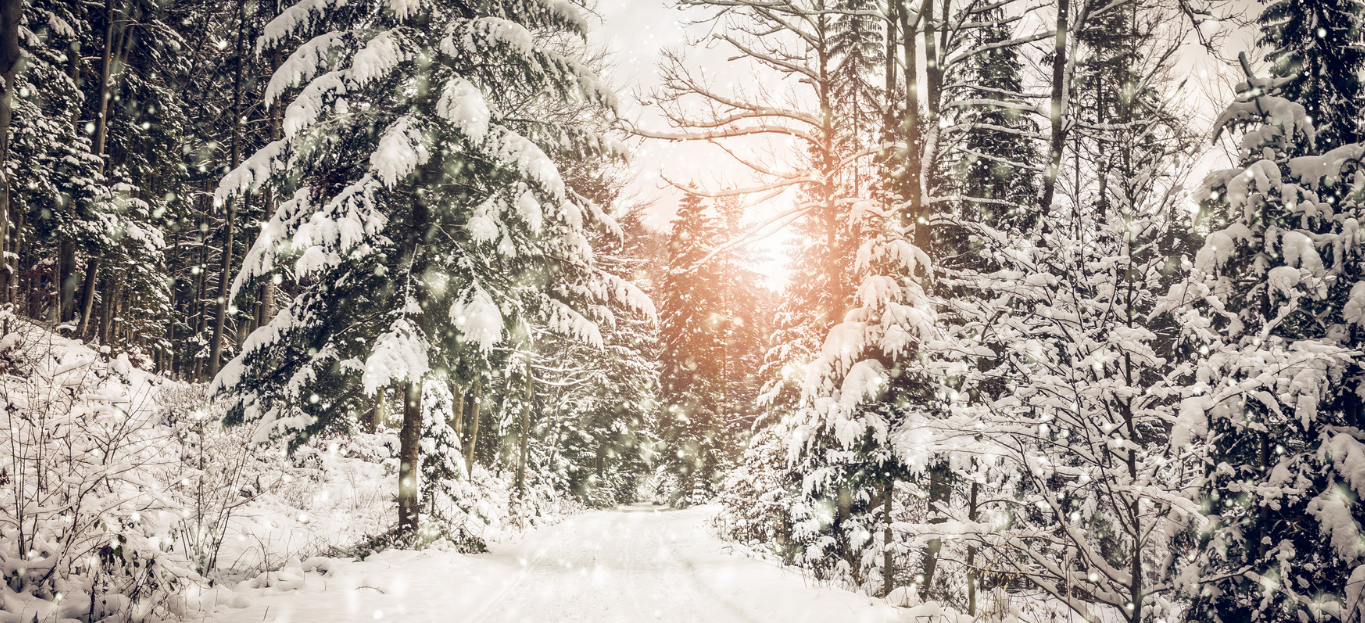This rectangular, horizontal photo captures a serene, snowy forest scene with remarkable detail. The main focus is a snow-covered path or road that bends off gracefully in the distance. Tall trees, possibly pine and other evergreen varieties, line both sides of the path. The trees are blanketed in snow, as are small bushes and patches of tall, dead grass protruding from the snow on either side. 

The scene is set during a snowfall, with snowflakes visibly falling, and the sun peeks through the trees just above the distant bend. This creates a warm, orange lens flare that cascades over the trees, suggesting either a sunrise or sunset. The predominant colors are the whites of the snow, the blacks and dark greens of the trees, the browns of the exposed grass, and the golden oranges of the sun's glow. This image, devoid of any textual elements, exudes a tranquil, winter atmosphere, highlighted by the contrasting hues and the subtle interplay of natural light.